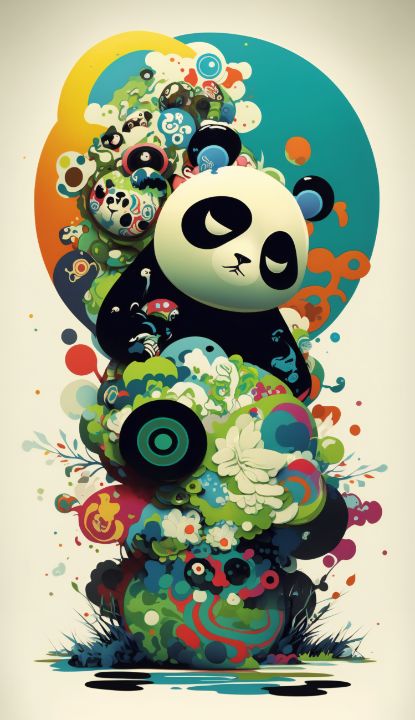This vibrant and whimsical illustration depicts a sad-looking panda with its head tilted slightly to the right, eyes closed, and mouth downturned. The panda's face is predominantly white with black patches around its eyes, and it has blue-tinted black ears. The upper body is black, while the lower body transitions into a myriad of colors, swirls, and circular floral patterns.

Behind the panda's head is a large, multicolored circle with a turquoise right half and a yellow-orange left half. This circle is filled with smaller circles resembling buttons and flowers in various hues, including blues, whites, blacks, pinks, and reds. These detailed patterns extend down to the lower part of the image, blending into a collection of colorful circles with floral prints, featuring green, turquoise, pink, and red shades.

The entire scene sits on an off-white background with a depiction of blue and black puddles and greenish grass-like elements at the bottom, adding a natural and somewhat abstract environment to this captivating artwork.